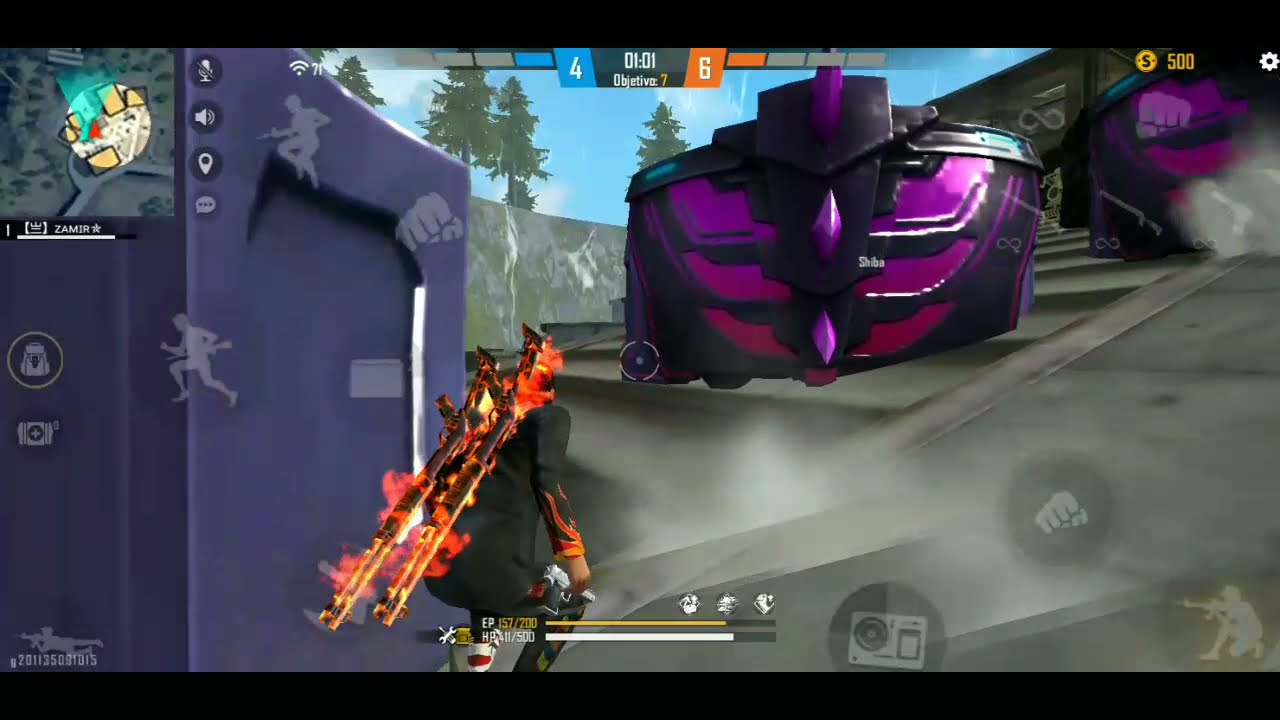In this detailed video game scenario screenshot, the player-controlled character is positioned in a third-person view with their back facing the camera, crouched next to the side of a large, blue metal container which resembles a dumpster. The character is outfitted in a black suit with flame designs creeping up the right sleeve of their long-sleeved shirt, adding a striking visual element. Slung across their back are two long guns, both exhibiting a vivid graphical effect of being on fire.

The screen's heads-up display (HUD) information is prominent, featuring a scoreboard at the top that indicates the blue team has 4 points while the orange team leads with 6 points. There is also a countdown timer visible, which reads 01:01. To the left of the screen, part of the scene includes a big purple structure that looks somewhat like a dumpster, with a box featuring a black and purple design along with a circular white and brown pattern, red spots, and some dark brown and white squares next to it. In the background, the sky and a couple of trees can be seen, adding further to the game's environment.

On the right side, there's a large stone wall with a sleek, purple sports car driving towards the screen. Beyond this car, a brown building with steps can be seen, with reflections subtly captured on varying surfaces. The ground beneath the purple car is gray, intersected by a long gray step running across the middle of the image. Also on the screen are various game control buttons, including a crouch button, a camera button, a fist button, a run button, a backpack button, and health bars labeled EP and HP at the bottom, which are standard in mobile gameplay. The landscape features alien-like barrier structures on what appears to be a hill, framing the player character’s hidden, tactical stance.